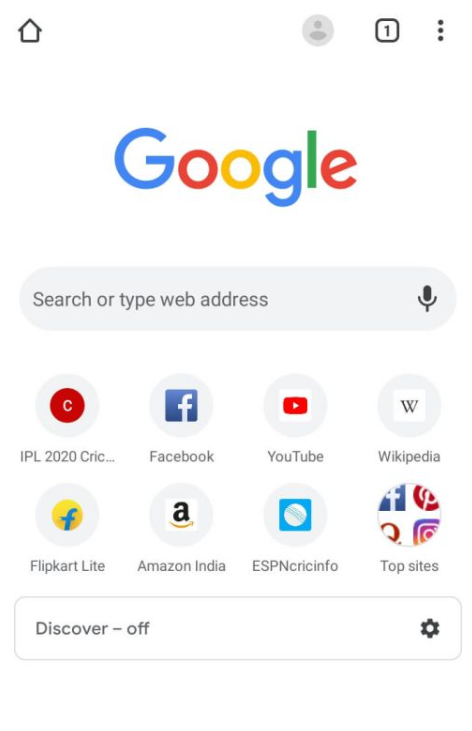The image features a Google search page displayed against a white background, resembling a person's home page with favorite websites shown as icons beneath the search bar. In the upper left-hand corner, there is a black-outlined house shape representing the home button. On the upper right-hand corner, a grayed-out profile icon is visible next to a box with the number '1' indicating the number of open tabs, and a vertical three-dot icon signifying additional options.

Centrally situated is Google’s iconic logo, featuring blue and red Gs, a red first O, yellow second O, and green L. Below the logo, a grey search bar reads “Search or type web address” and includes a microphone icon for voice search options. The bottom part of the page mentions "Discover is off" next to a cogwheel icon for settings.

Highlighted are eight favorite website icons: IPL 2020 CRIC, Facebook, YouTube, Wikipedia, Flipkart Lite, Amazon India, ESPN, and Crick Info, culminating with a summary section labeled "Top Sites."